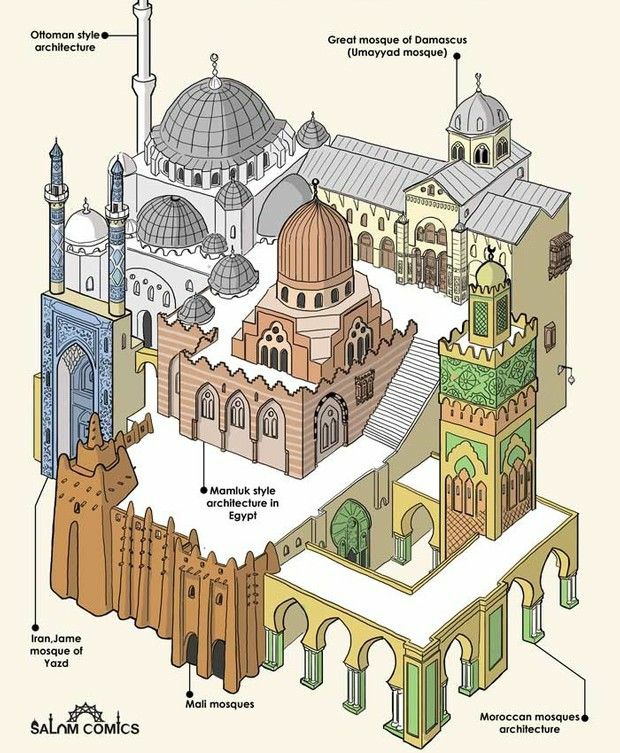This detailed axonometric illustration showcases various notable examples of Islamic architectural styles, each labeled with identifying text. In the top left corner, there's an Ottoman-style structure characterized by its dome and tower. Adjacent to it, towards the right, is the Great Mosque of Damascus, also known as the Umayyad Mosque. In the middle of the image, a castle-like structure represents Mamluk architecture from Egypt, featuring a dome as well. On the lower left, the Iran Jame Mosque of Yazd is depicted with its distinctive tall blue towers and gate. Below the central structure, a segment tagged as 'Mali Mosques' highlights walls with traditional buttresses. Finally, at the bottom right, the Moroccan mosque architecture is represented by a vibrant colonnade with a tower displaying a mix of pink and green hues. The illustration, appearing as if sourced from an encyclopedia or architectural magazine, employs 2D axonometric projection to present these varied designs, each precisely annotated to convey the rich diversity within Islamic architecture. The image also bears the 'Salam Comics' icon, featuring an Islamic dome and Ottoman-style towers integrated into the lettering.